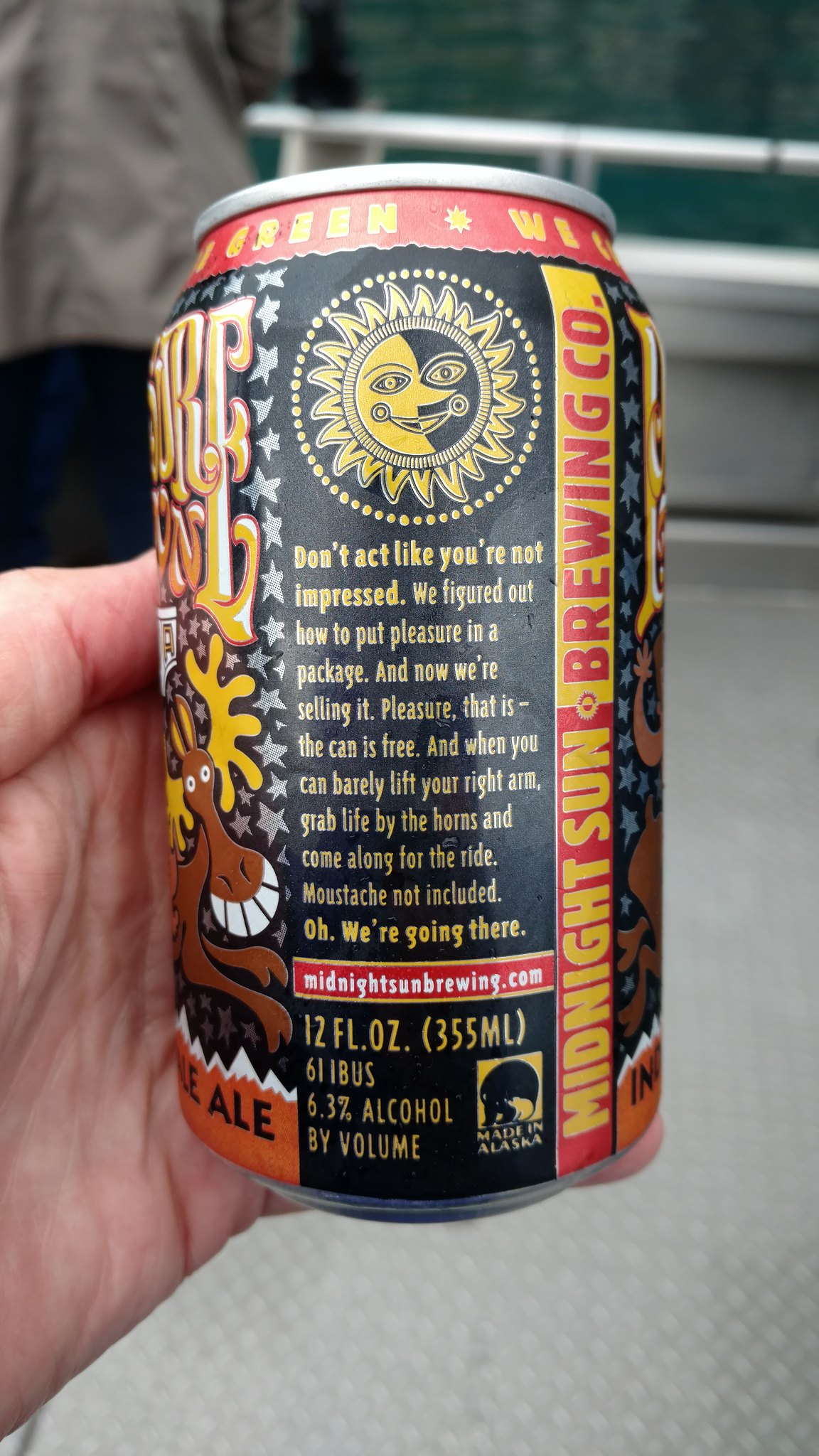This image features an aluminum can of Midnight Sun Brewing Company’s ale. The can is adorned with a vibrant red and yellow strip running vertically along its side. At the top of the can, there is a round emblem of a sun, split into yellow and black halves. The can bears the slogan, "Don't act like you're not impressed. We figured out how to put pleasure in a package, and now we're selling it. Pleasure that is, the can is free." An additional quirky message encourages, "When you can barely lift your right arm, grab life by the horns and come along for the ride, mustache not included. Oh, we're going there." Adding to its quirky design, there's an illustration of a moose with yellow ears. Finally, the word "ale" is prominently displayed at the bottom of the can.